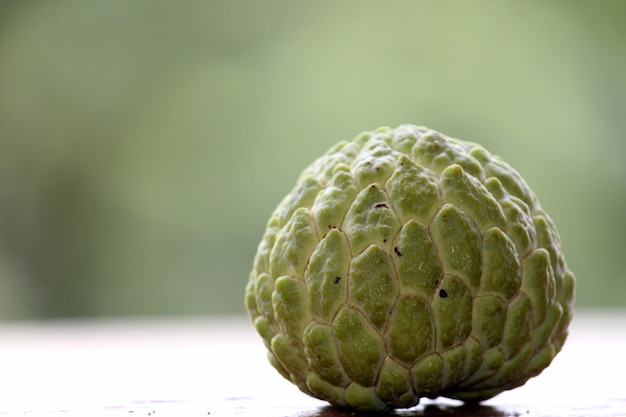This color photograph, taken outdoors in landscape orientation, prominently features a single sugar apple situated slightly off-center towards the bottom right of the image. The fruit, resting on its broad end with its tapered end pointing upwards, exhibits a distinct scaly texture. Each scale is primarily green, gradating to lighter shades, verging towards tan around the edges. Covering approximately 30 to 40 percent of the image, the fruit’s detailed surface is highlighted by its shingled appearance, reminiscent of an upside-down apple. The sugar apple sits atop a flat, off-white surface that stretches across the bottom quarter of the photograph. The background, filled with muted greens and browns, remains blurry, making it difficult to discern the exact outdoor setting.